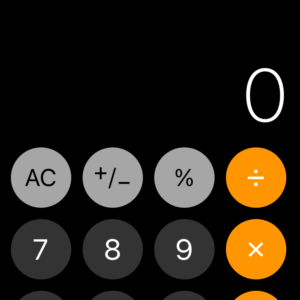The image showcases a mobile screenshot of a calculator app with a sleek black background. At the top right corner, a white arrow icon is prominently displayed. Below the arrow, various symbol buttons are arranged in circles. The AC (All Clear), plus/minus, and percent symbol buttons are light gray. The division and multiplication symbol buttons stand out in orange. The numbers seven, eight, and nine are in dark gray circles. Although the image is cropped, you can see hints of additional buttons in more dark gray and orange colors below the visible area.